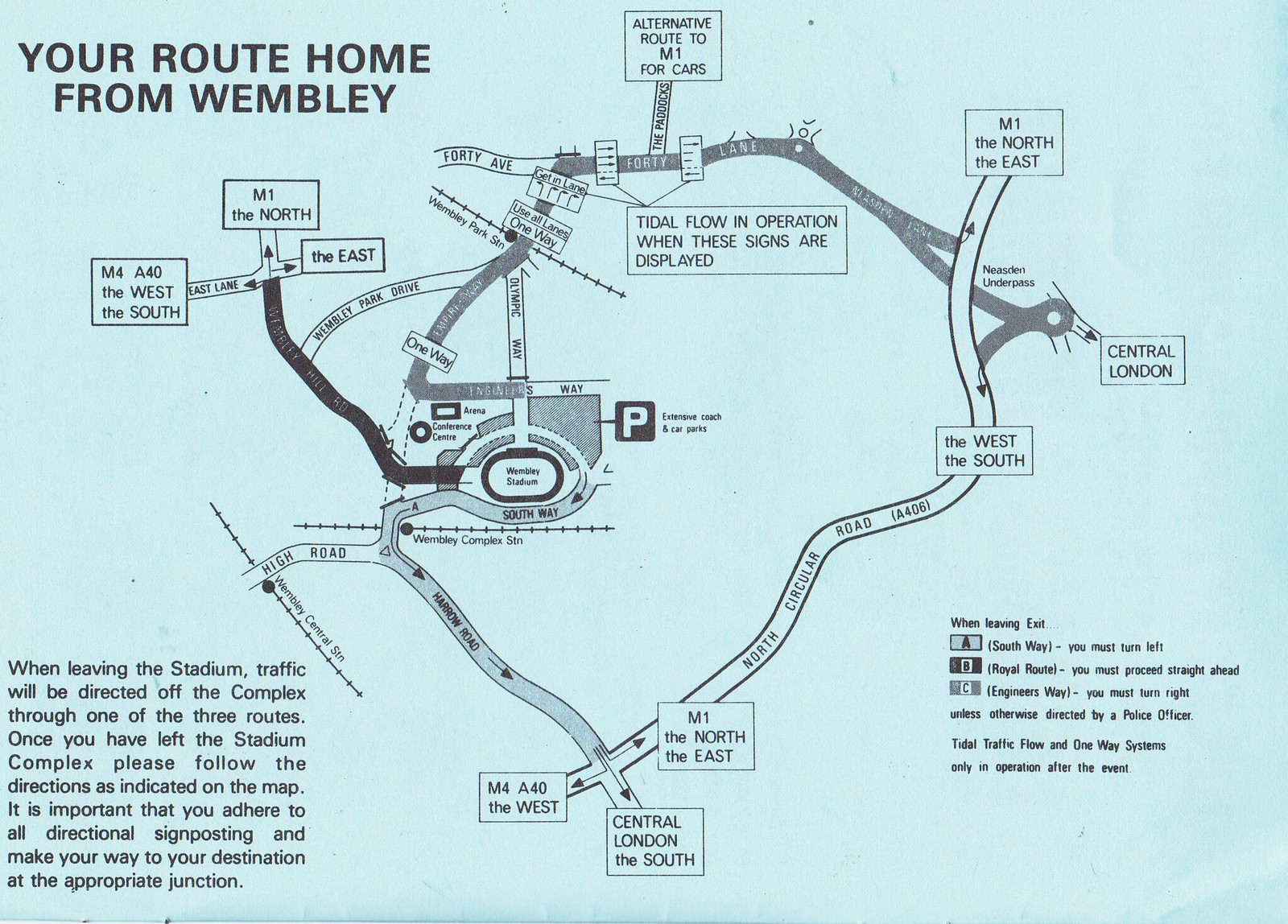This image is a detailed map, printed on light blue paper, depicting the route home from Wembley Stadium. The text on the map is primarily in black with varying shades of darkness, and specific directions are highlighted in boxed labels. In the bottom left corner, there is an explanation that reads: "When leaving the stadium, traffic will be directed off the complex through one of the three routes. Once you have left the stadium complex, please follow the directions as indicated on the map. It is important that you adhere to all directional signposts and make your way to the destination at the appropriate junction." The map prominently features Wembley Stadium and its parking area, and it outlines various routes to central London, the southwest, the south, and the M1 for northern destinations. Arrows indicate the directions to be followed, making clear the paths for drivers to exit the Wembley complex and reach their homes.